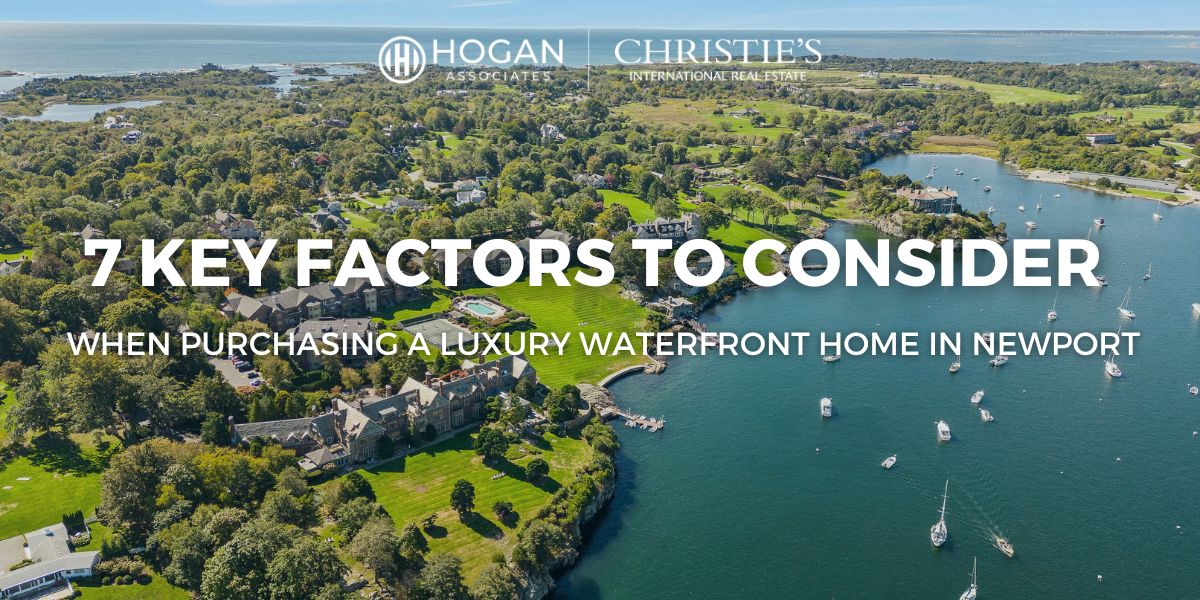The advertisement features a horizontally aligned, rectangular aerial photo captured during the daytime, showcasing a picturesque coastal landscape. The scene is dominated by the clear blue horizon of the ocean at the top of the image, transitioning into lush green land in the foreground. The land is richly covered with beautiful green grass, dense clusters of trees, and a smattering of impressive large homes or buildings. A smaller, greenish-gray body of water curves from the lower right through the middle, dotted with at least 20 white boats. Centered at the top of the image, a logo features a white circle with an 'H' inside, accompanied by the text "Hogan Associates" and "Christie's International Real Estate" to its right. Bold, white, capitalized letters across the center of the image read, "SEVEN KEY FACTORS TO CONSIDER," and below that, in smaller white capital letters, "WHEN PURCHASING A LUXURY WATERFRONT HOME IN NEWPORT."